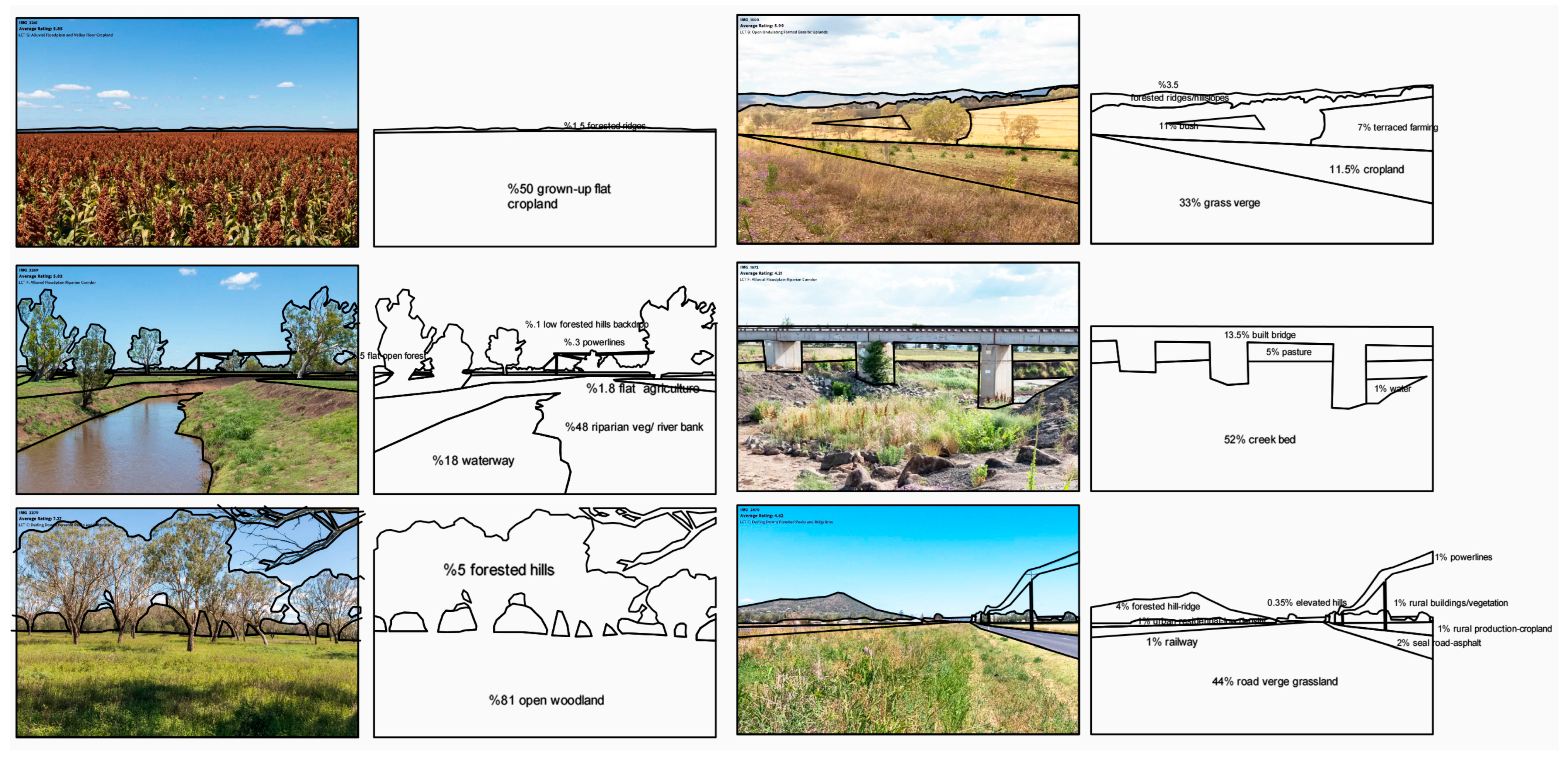The image features a composite layout of 12 illustrations arranged in four sets of three, where each set displays a progression from colored scenery to its corresponding line drawing. On the left side, each set begins with three color-rich illustrations depicting various natural and rural landscapes, primarily showcasing fields with significant hues of brown, green, and blue. Each color scene is paired with an adjacent black and white line drawing that outlines the topographical features and annotations detailing the proportion of different elements in the scene, such as "50% grown-up flat cropland" or "30% grass verge".

For instance, the first group features a picturesque cornfield stretching to the horizon, with blue skies above. The accompanying line drawing highlights the topography, revealing insights like the extent of the cropland. Another group portrays a highway bordered by grassy areas and distant mountains, marked by telephone poles. The line drawing deconstructs the scene, indicating the spatial distribution of grassland, roadway, and mountains.

This systematic combination continues through all four sets, providing detailed visual and descriptive narratives of fields, bridges, trees, water bodies, and train paths, effectively merging photographic elements with instructional line illustrations to convey the landscape's composition and land use.